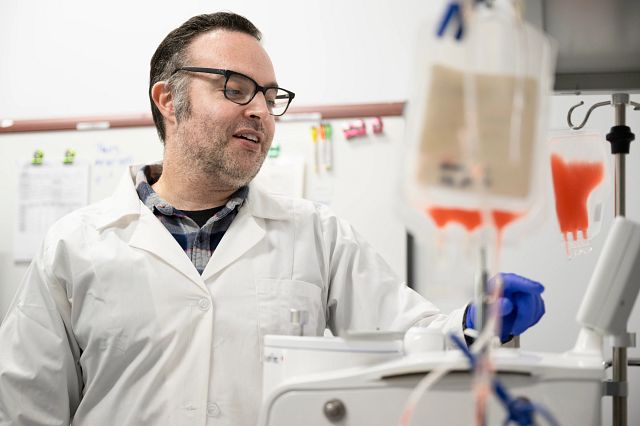The photograph captures a detailed scene inside a medical or laboratory setting, featuring a middle-aged male worker who could be a doctor, scientist, or lab technician. He is positioned on the left side of the image, wearing a white lab coat over a black and white flannel shirt, which in turn covers a black t-shirt. He has short, dark hair with gray at the temples, and sports black-rimmed glasses along with a short gray beard. His hands are gloved in blue surgical gloves. To his right, he is interacting with or examining a white machine, its specifics indistinguishable. Nearby, an IV stand holds a bag filled with white liquid, and in the background, another IV bag contains an orange liquid. Behind him, a whiteboard with writing and clips, as well as a white wall and possibly a window, are visible, providing context to the clinical environment. His pens peek out from the pocket of his lab coat, further indicating his professional setting.